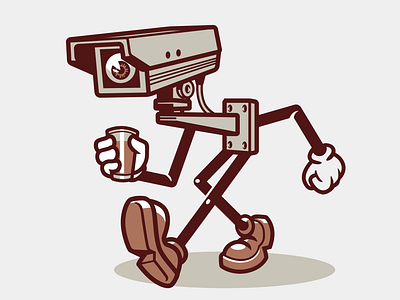The image depicts a cartoon, clipart-style anamorphic CCTV camera. The upper half of the body resembles a horizontal security camera with an eyeball where the lens would typically be, giving it a lifelike appearance. The neck and head are part of the mounting bracket designed to resemble a shoulder and torso. The camera has stick figure-like arms ending in white gloves reminiscent of Mickey Mouse gloves. One arm is akimbo while the other is extended, holding a glass of orange liquid, potentially orange juice. Its stick-like legs, starting from the chest area, are dressed in bulky brown cartoonish shoes, with one leg bending and the other stretching out, creating a slouching posture. The entire scene sits on a light gray background, with a subtle shadow circle under the figure to suggest its presence.